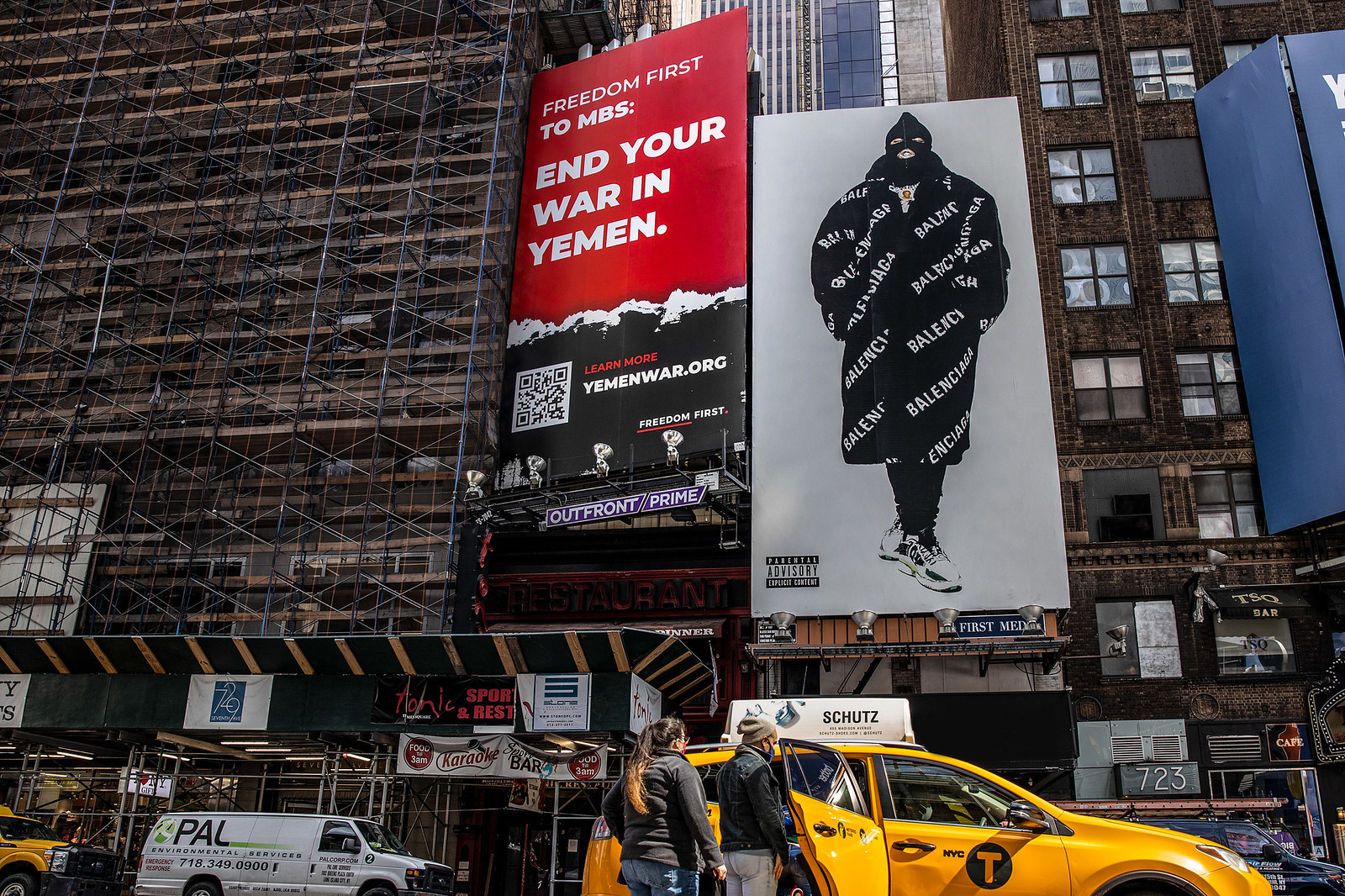In this urban scene, a bustling city street features striking protest posters plastered on the side of a building. The most prominent sign is a large, bold poster in red, white, and black, emblazoned with the message "Freedom First to MBS, End Your War in Yemen." Below this call to action, a scannable QR code offers further information via YemenWar.org. Adjacent to this poster is another impactful image: a stark, white backdrop showcases a figure wearing a ski mask and a distinctive coat, with the words "Both Valencia" emblazoned across the front. This imagery is strategically positioned to catch the eyes of passersby, contrasting sharply with the grey urban surroundings. 

In the foreground, a classic yellow taxi cab navigates the street, accompanied by several work vans, emphasizing the everyday hustle and dynamic energy of the city. The detailed tableau captures a moment of protest and activism amidst the backdrop of daily urban life.